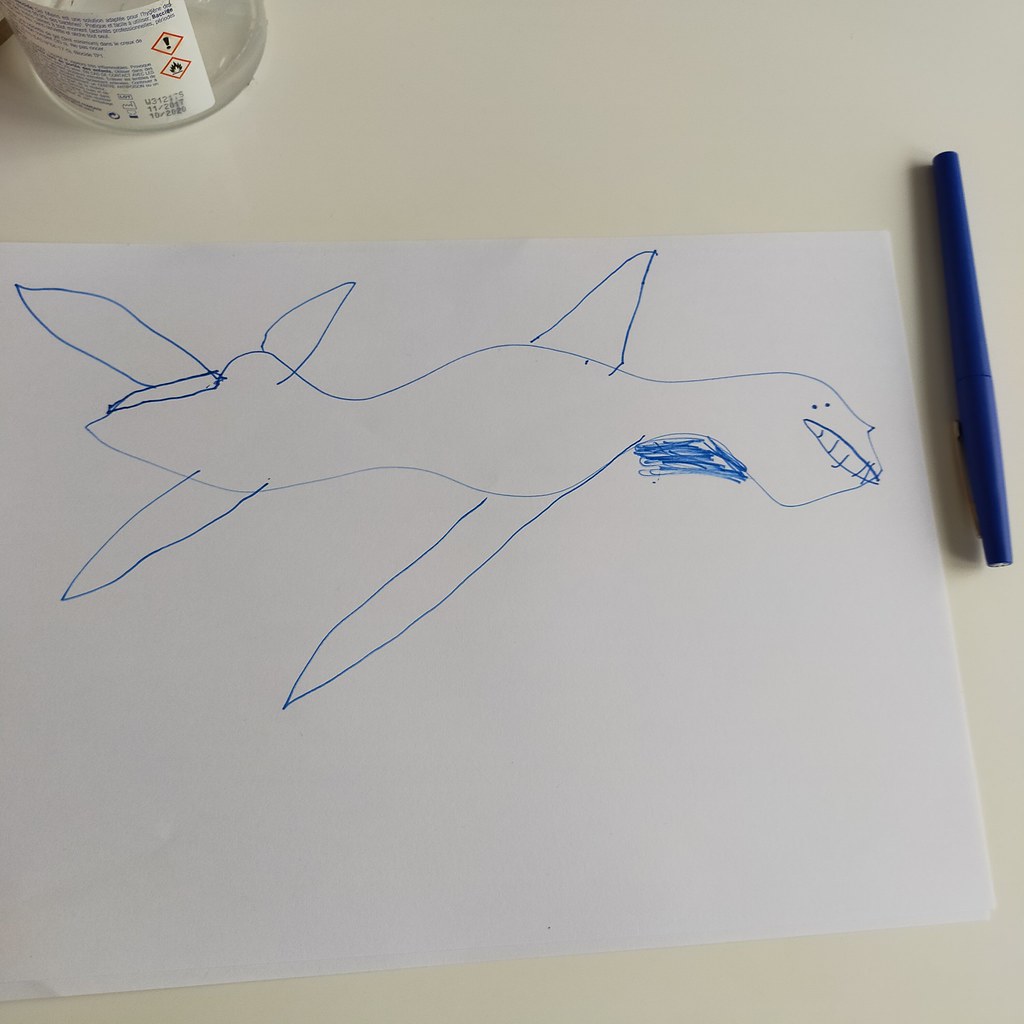In this image, a detailed drawing created with a blue thin-tipped marker is prominently featured on a white piece of paper, which is laid out on an off-white table. In the upper left corner of the table sits a jar with its label facing towards the viewer. To the right of the paper, the blue marker used for the drawing is visible, casting a shadow along its left side. The artwork itself depicts what appears to be a marine creature, likely a shark or a dolphin, oriented towards the right. The creature has a closed mouth lined with teeth and two dot eyes. Below its neck, there is an area of dark blue scribbles, and the body is detailed with four side fins and one additional fin protruding from the back.